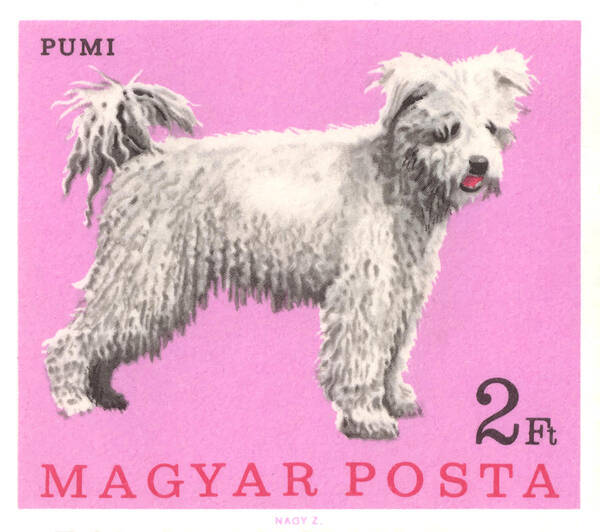The image is a photograph of a postage stamp, set against a pink or purple background, featuring a white dog with shaggy fur, black eyes, and a black nose. The dog is in profile with its body facing left, tail up like a pom-pom, and head turned slightly toward the camera, showing its pink tongue and its white teeth. The text "PUMI" is in the top left corner in black, while "2FT MEG YA POSTA" appears in a larger red text at the bottom, with additional letters "NAGYZ" outside the stamp. The dog appears to be leaning forward, with its back paws slightly off the ground.